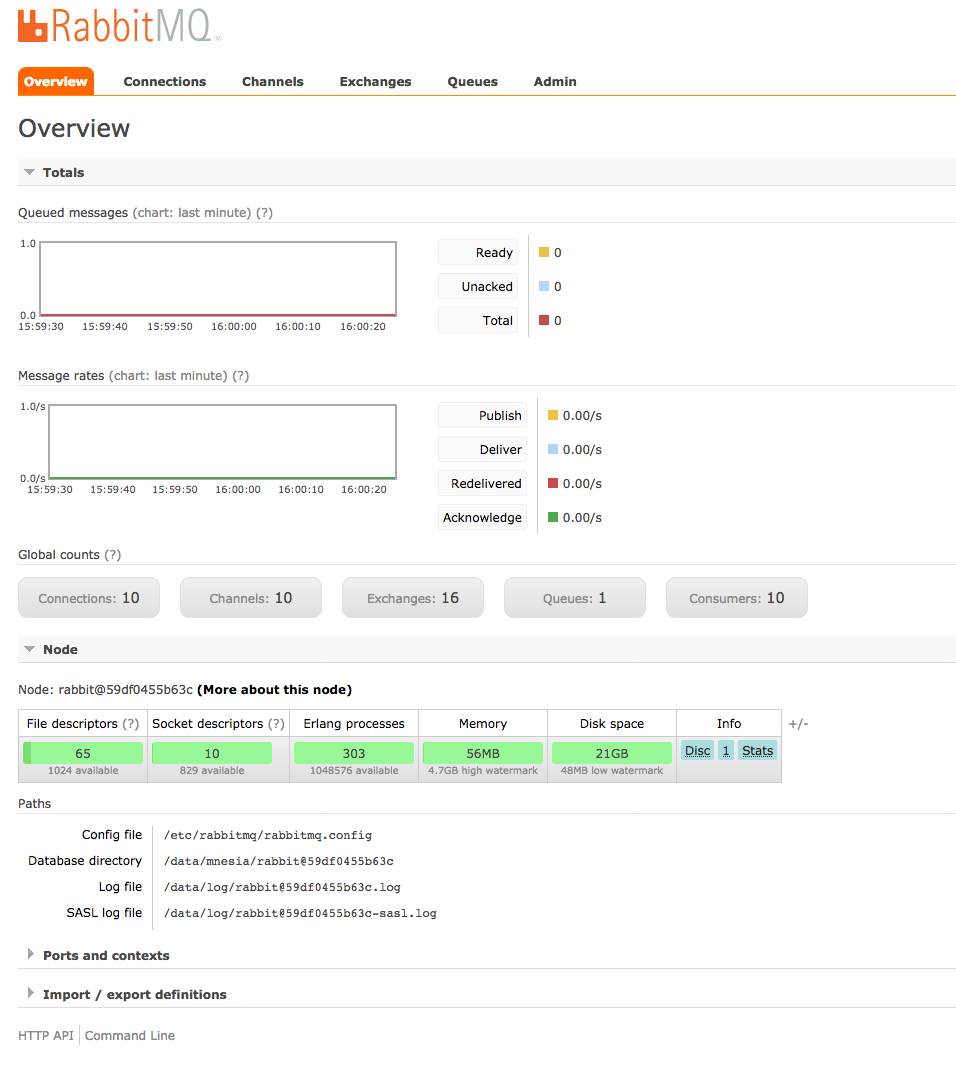This screenshot showcases the RabbitMQ application interface, featuring a logo on the left depicting a rabbit composed of pixelated blocks. Beneath the logo, various tabs and categories are displayed, with the current tab being "Overview," highlighted with an orange overlay. The other tabs include "Connections," "Channels," "Exchanges," "Queues," and "Admin."

The Overview tab provides an extensive array of data and configuration options, presented through a mix of numbers, text, charts, buttons, and input boxes. It's not immediately user-friendly due to the density of information and options available. Key sections on the Overview tab include nodes information, configuration files, database settings, directory paths, log files, SASL log files, along with other detailed categories such as ports, contexts, imports, and export definitions.

Moreover, there is a reference to an HTTP API and command line tools used for managing and coding within the RabbitMQ environment. The current state of the chart on this tab shows many fields with zeros, indicating that it hasn't been populated with data yet. This detailed view is just one part of the comprehensive Overview tab within RabbitMQ's interface.